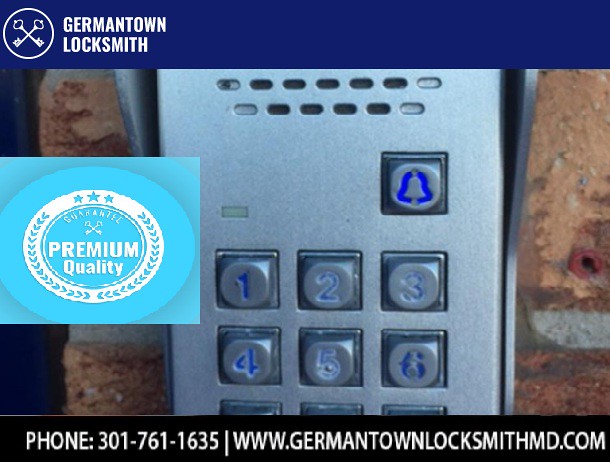This advertisement flyer for Germantown Locksmith showcases a central image of a gray stainless steel keypad door lock with a blueish call box, featuring number buttons from 1 to 9 and an alarm button. The scene is set against a red brick wall that frames both sides of the image. The image utilizes landscape orientation.

At the top of the flyer, a blue horizontal banner displays the text "Germantown Locksmith" in bold white letters, with a white circular logo depicting two crossed keys to the left. Positioned mid-left, a light blue shield-like rectangle inscribed with "Premium Quality" adds visual detail to the design.

A black strip runs along the bottom of the flyer, with the company's contact information: "Phone: 301-761-1635" and "www.germantownlocksmithmd.com" presented in striking white text. The flyer blends photographic realism with graphic design elements and typography, effectively advertising the professional services of Germantown Locksmith.